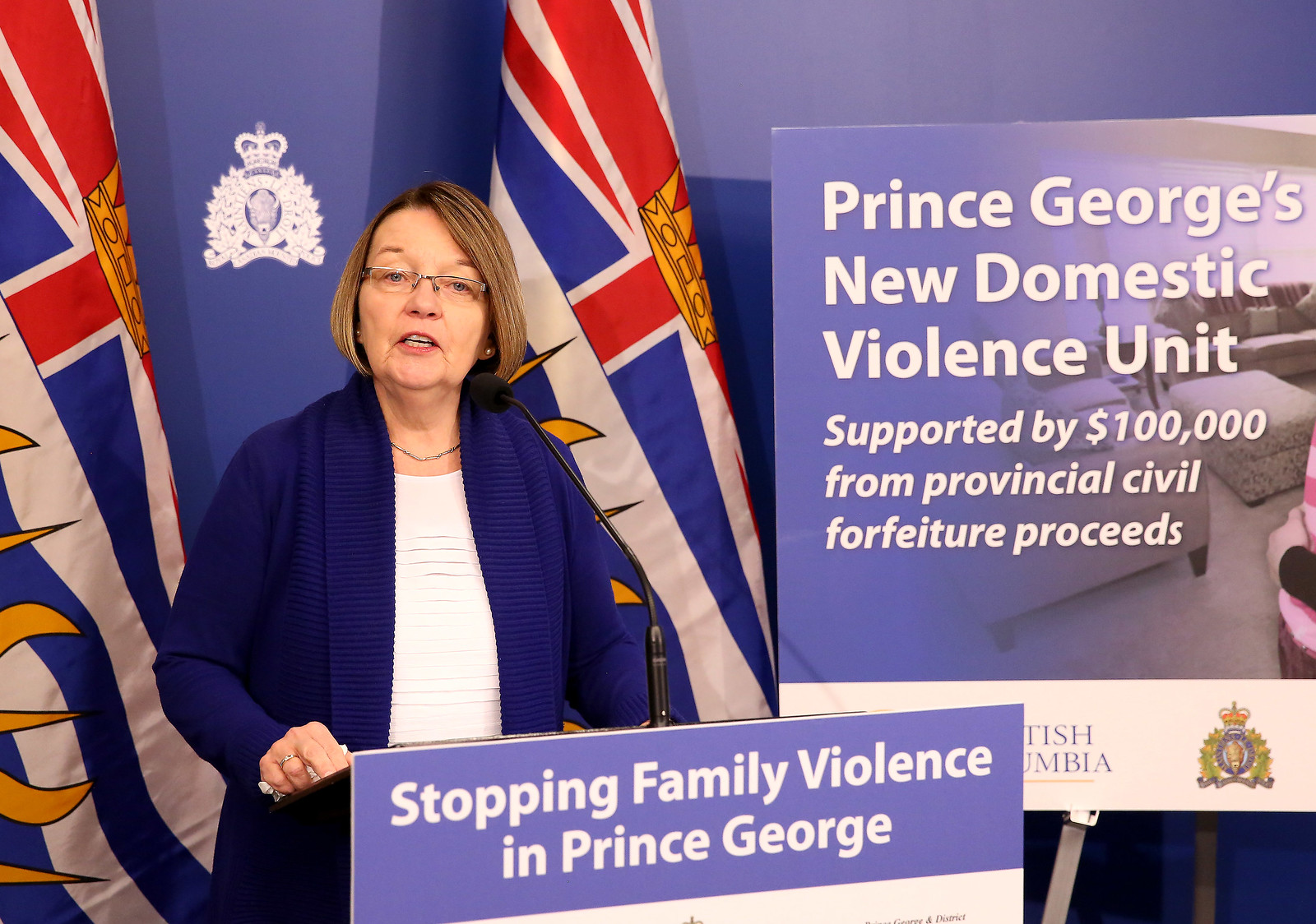In this image, a British Columbia politician is delivering a heartfelt speech about stopping family violence, part of a campaign supported by $100,000 from provincial civil forfeiture proceeds. The backdrop features poster boards and banners showcasing the British Columbia emblem and related information. The politician, a woman around 51 years old, exudes an approachable and sincere demeanor. She is dressed in a blue cardigan, accessorized with rings, glasses, and earrings. The setting seems spontaneous and relaxed, suggesting a community-focused event. Despite the serious topic, the moment captures the politician's genuine concern and commitment to the cause.